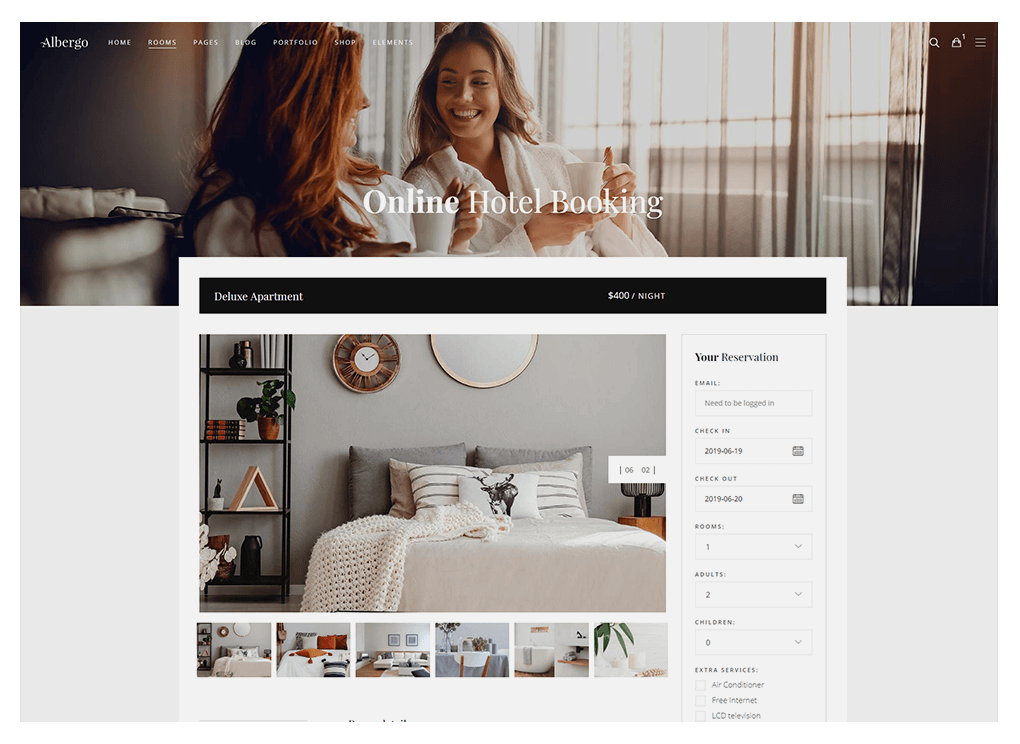The image appears to be a screenshot from an online hotel booking website. In the upper left-hand corner, the brand logo is visible with the name "Albergo." Adjacent to the logo is a navigation menu featuring categories such as Home, Rooms, Pages, Blog, Portfolio, Shop, and Elements, with 'Rooms' underlined in white.

The background image showcases two women in a hotel room, both smiling and holding white coffee cups. The woman on the left has long, reddish hair and is looking at the blonde woman on the right, whose face is mostly visible. Both women are dressed in white bathrobes.

Beneath the image, in a white information box, the text "Deluxe Apartment" is on the left, and "$400 a night" is on the right. The room description includes a picture of a bed adorned with six pillows and a decorative cushion, a black stand with four shelves, a wheel-shaped clock, and a circular mirror above the central pillows. Six thumbnail images present additional views of the apartment, including different angles of the bedroom, the living room with a couch, a dining area with a table, a bathroom with a white bathtub, and a white bathroom counter adorned with a green plant.

To the side of the images, a column titled "Your Reservation" details booking information. The section includes an email prompt requiring login, check-in and check-out dates (2019-06-19 to 2019-06-30), and drop-down menus for the number of rooms, adults, and children. Extra services available for selection, but not currently checked, include air conditioning, free internet, and an LCD television.

Overall, the screenshot serves as a detailed representation of an online hotel booking page, showcasing room options and reservation details.